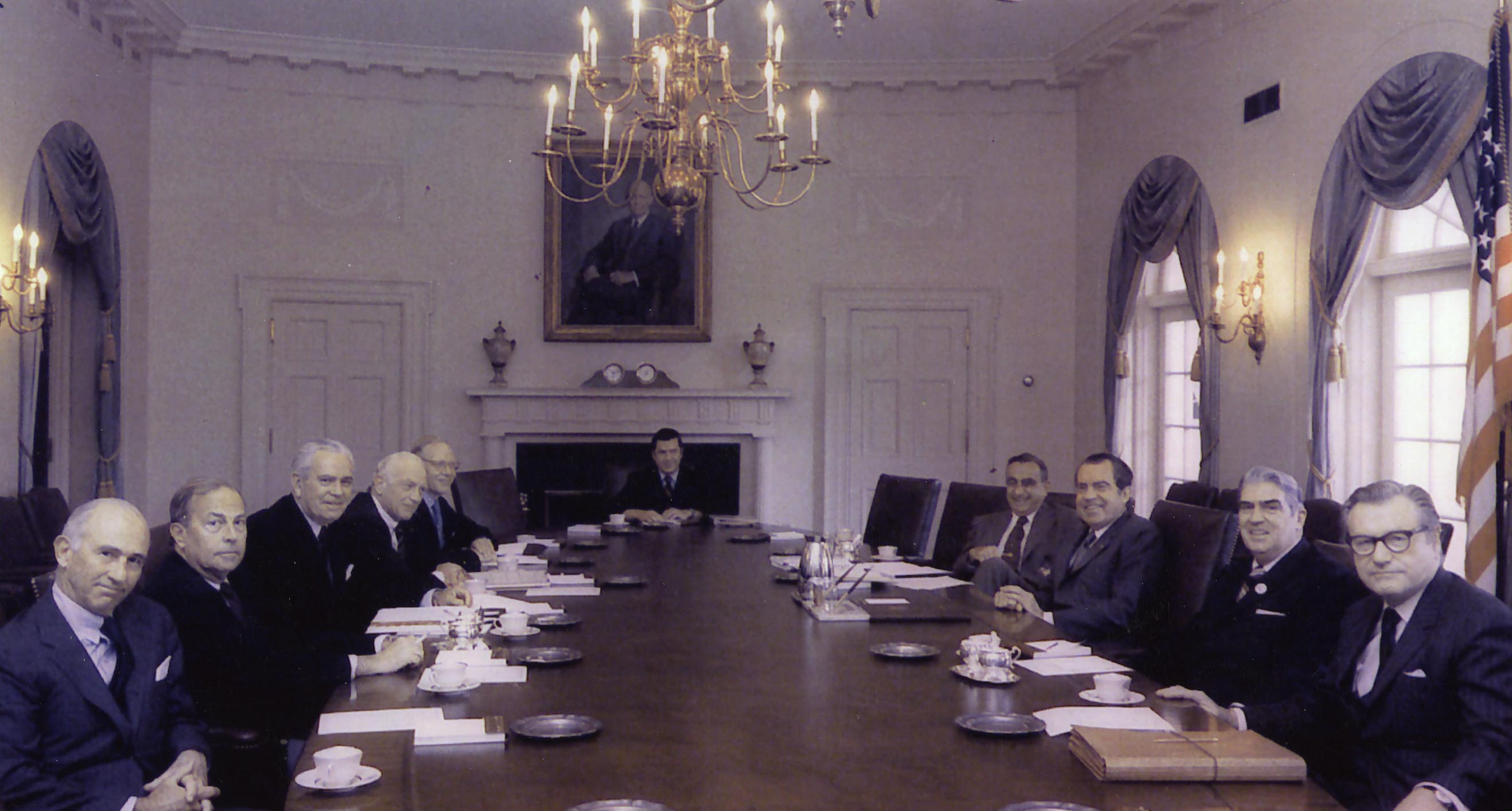The photograph depicts President Nixon meeting with his cabinet or advisers around a large, oval wooden table. Nixon is positioned on the right side of the table, joined by three other men. Opposite them, on the left side, sit five men, most wearing dark suits, with the exception of the man at the far end who is in a blue suit. Each individual has various documents, teacups, and silver trays in front of them, indicating an important meeting. A man in a dark suit is seated at the far end of the table. The setting is unmistakably the White House, evidenced by the white walls, a portrait of President Eisenhower hanging above a fireplace, two doors to the left and right of the back wall, and an American flag positioned in the back right corner. The room is adorned with a chandelier and additional light fixtures that resemble candles, and features arched windows with blue valances and side curtains. Several empty chairs are present around the table, hinting at a potentially larger gathering.